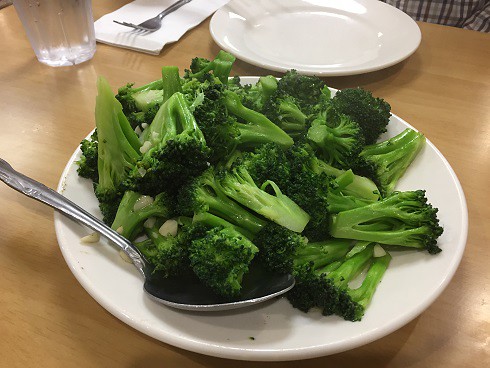The image captures a dinner scene set on a light brown wooden table. The focal point is a white dinner plate laden with bright green broccoli, softened and likely steamed, adorned with a dark green leaf on top. A silver serving spoon holds a portion of the broccoli at the bottom of the plate. Beside this, in the upper left corner, stands a clear glass of cold water, evidenced by the beads of condensation on its surface. Adjacent to the glass, there is a white rectangular napkin neatly placed with a clean silver fork on top of it. In the background, another plate sits empty in front of a person wearing a tan, brown, and white plaid shirt, hinting at a shared dining experience, perhaps in a restaurant setting.